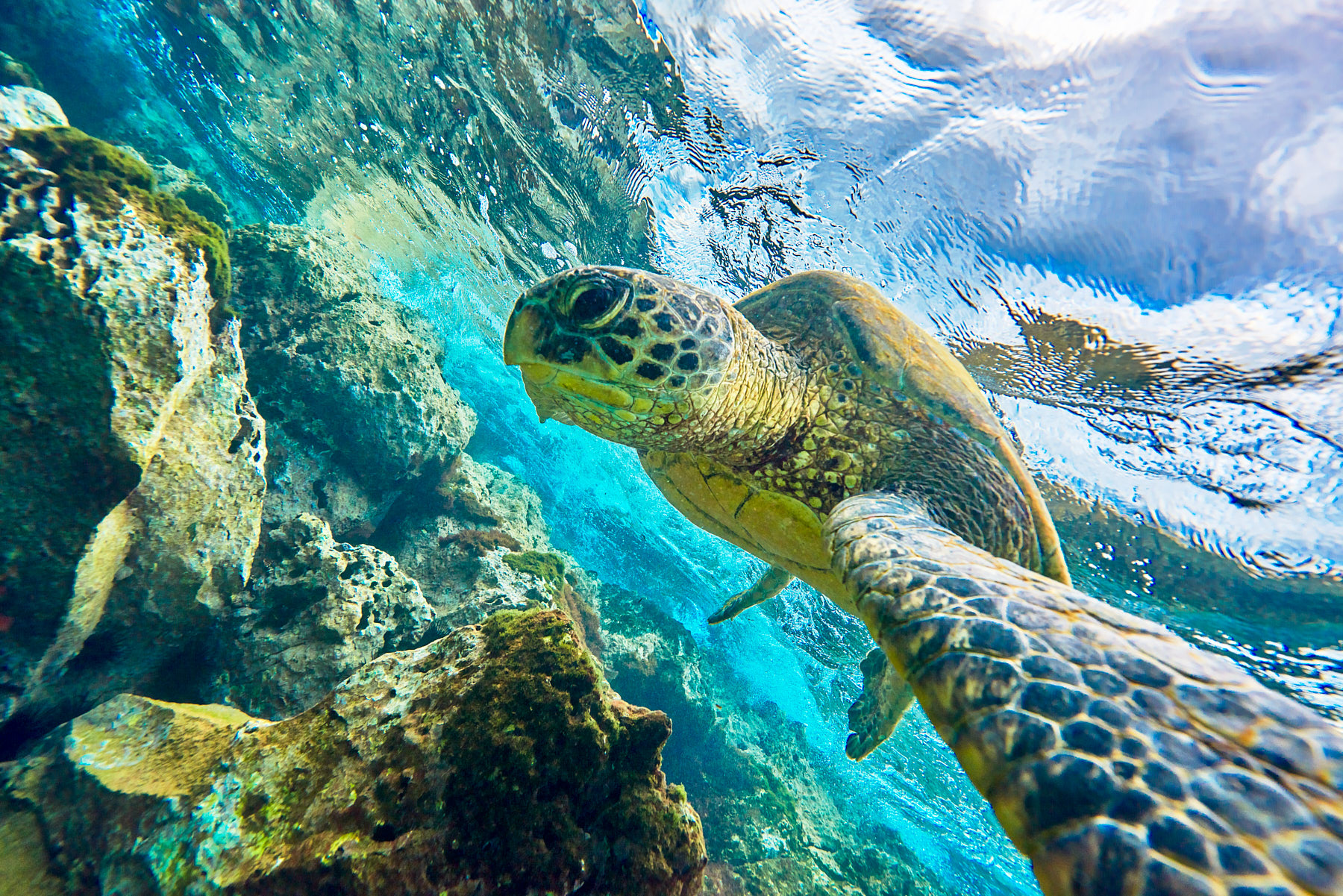This underwater photograph captures a serene scene of a sea turtle swimming gracefully among moss-covered rocks. The turtle, with its yellow and black patterned shell, extends its flippers as if elegantly navigating the clear, tropical waters. Its large, dark eyes seem to curiously inspect the surroundings, contributing to the humorous illusion that the turtle might be taking a selfie. Above the turtle, the surface of the water reflects the blue skies and occasional clouds, while the sun's rays penetrate to illuminate the setting. The rocks, adorned with greenish moss, likely provide a source of food for the turtle. The overall color palette predominantly features hues of blue, mingled with the greens of the moss and the contrasting colors of the sea turtle, creating a vivid snapshot of a warm, tropical underwater environment.